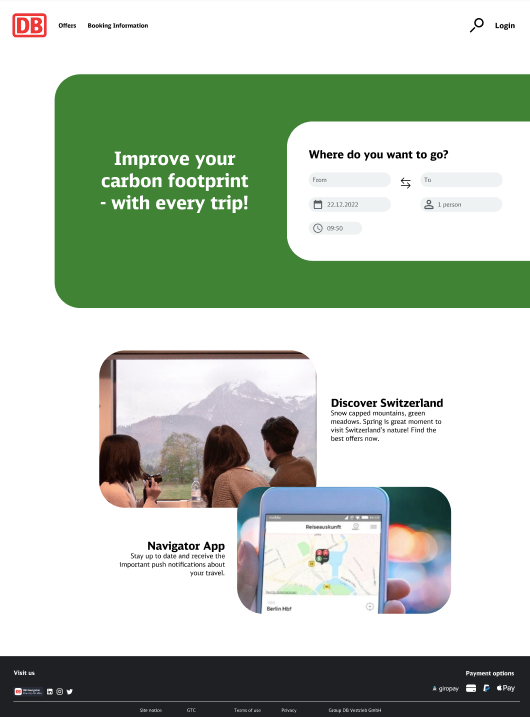This screenshot from a travel website has a clean white background. In the upper left corner, there is a red-lined rectangle containing the red, capitalized letters "DB." To the right, small black text reads "Offers" followed by booking information. In the upper right corner, there is a black magnifying glass icon next to the word "Login."

Below this, a large green rectangle with rounded corners stretches across the screen. In the left-center of the green rectangle, white text states, "Improve your carbon footprint with every trip." Inside this green rectangle, on the right side, there is a white rectangle with rounded corners. This white rectangle contains a black text box where users can input their travel details, starting with "Where do you want to go." Below this header, there is an input field with the placeholder text "From" followed by directional arrows and the destination name. Beneath this, users can select travel dates, the number of travelers, and choose the time of travel.

Further down, there is a photo of three people looking out of a window, with a mountain visible in the background. The person furthest to the right is a male with short brown hair wearing a brown turtleneck shirt. In the center, there is a Caucasian female with long brown hair dressed in a light gray sweater. On the left, another Caucasian female with shoulder-length brown hair is wearing a white sweater. To the right of this group, bold text reads, "Discover Switzerland."

Below this section, there is an image of a hand holding a smartphone displaying a navigation app.